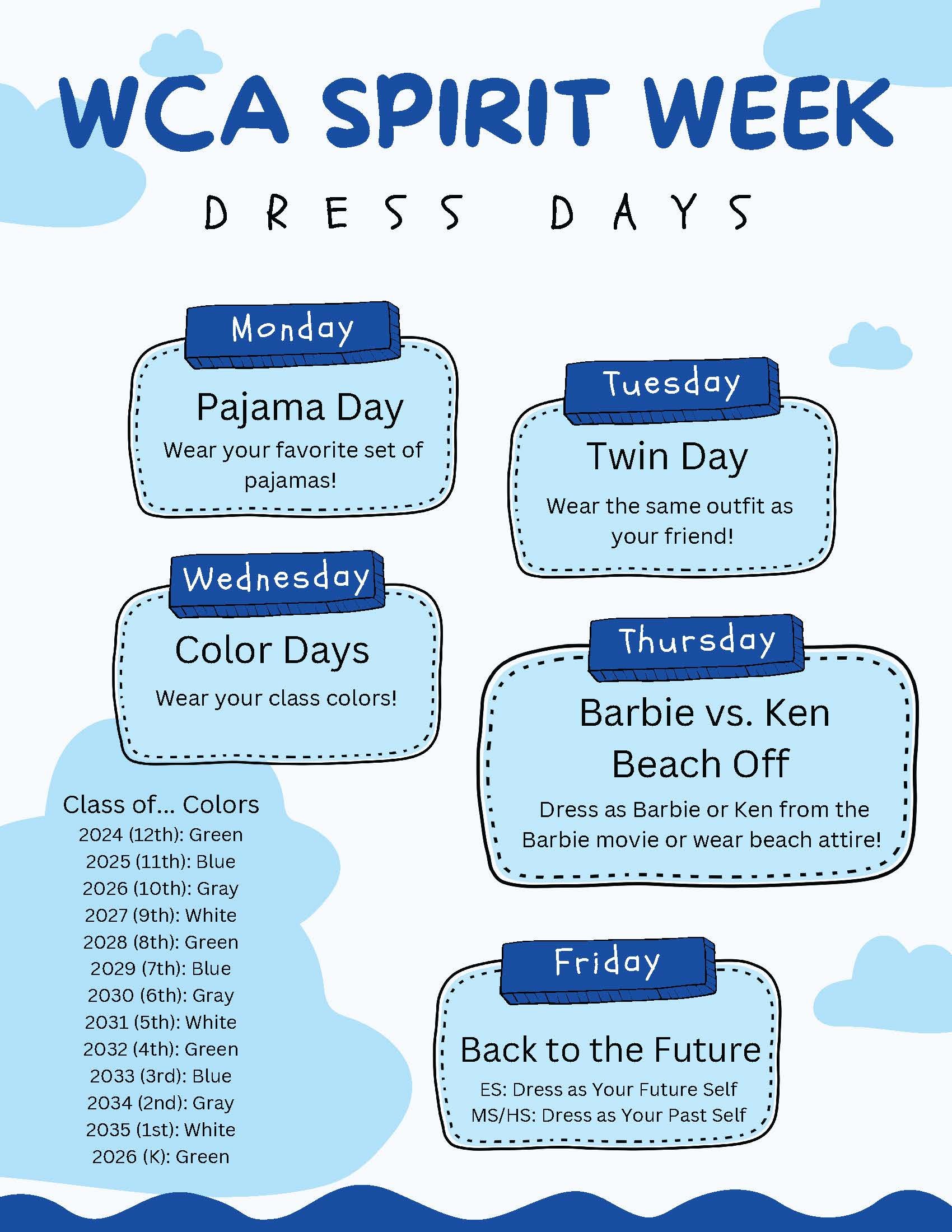This detailed infographic for WCA Spirit Week features a white background adorned with light blue clouds and a blue wave pattern along the bottom. The headline, "WCA Spirit Week," is prominently displayed at the top in blue sans-serif font, followed by "Dress Days" in a black handwriting-style font. Beneath, a sequence of curved rectangular boxes zigzags from the top left to the bottom right, listing the daily themes:

- **Monday:** Pajama Day—wear your favorite set of pajamas
- **Tuesday:** Twin Day—match outfits with a friend
- **Wednesday:** Color Days—each class wears their designated color
- **Thursday:** Barbie vs. Ken Beach Off—dress as Barbie or Ken from the Barbie movie or in beach attire
- **Friday:** Back to the Future—elementary students dress as their future selves, while middle and high schoolers dress as their past selves

In the bottom left corner, a section titled "Class Colors" details the assigned colors for each grade, spanning from the Class of 2024 to the Class of 2035, with an apparent typo replacing 2036 with 2026:

- 2024 (12th grade) - Green
- 2025 (11th grade) - Blue
- 2026 (10th grade) - Gray
- 2027 (9th grade) - White
- 2028 (8th grade) - Green
- 2029 (7th grade) - Blue
- 2030 (6th grade) - Gray
- 2031 (5th grade) - White
- 2032 (4th grade) - Green
- 2033 (3rd grade) - Blue
- 2034 (2nd grade) - Gray
- 2035 (1st grade) - White
- 2036 (Kindergarten) - Green